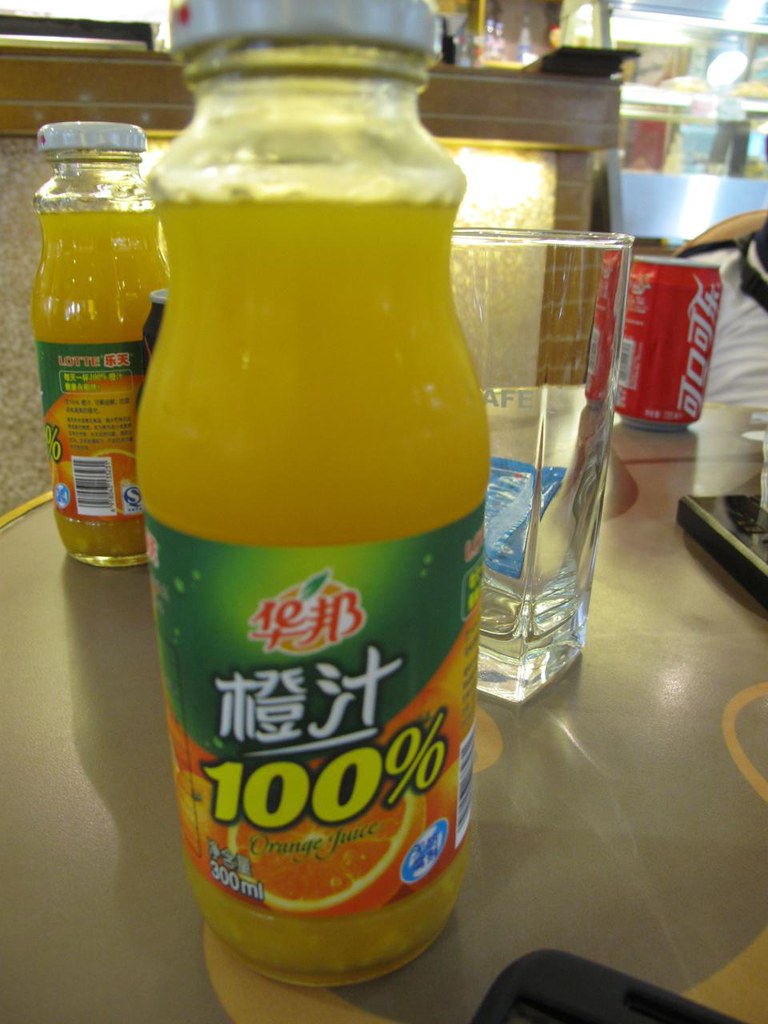This is a photorealistic image centered on a glass bottle of orange juice, likely taken in a restaurant or cafeteria setting. The bottle, about six to seven inches tall and holding 300 milliliters of liquid, features a wrap-around label with both English text and Asian characters, likely Chinese. The label is green on top and orange on the bottom, displaying "100%" in yellow outlined in black and "orange juice" in green lettering alongside a drawing of a sliced orange. The bottle has a white cap. Directly behind it is a square-shaped clear glass tumbler, empty, and to the right, a can resembling Coca-Cola with non-English text. To the left in the background, there is a second identical bottle of orange juice. The backdrop includes a stainless steel refrigerator and various brown and yellow drawings on the tabletop.